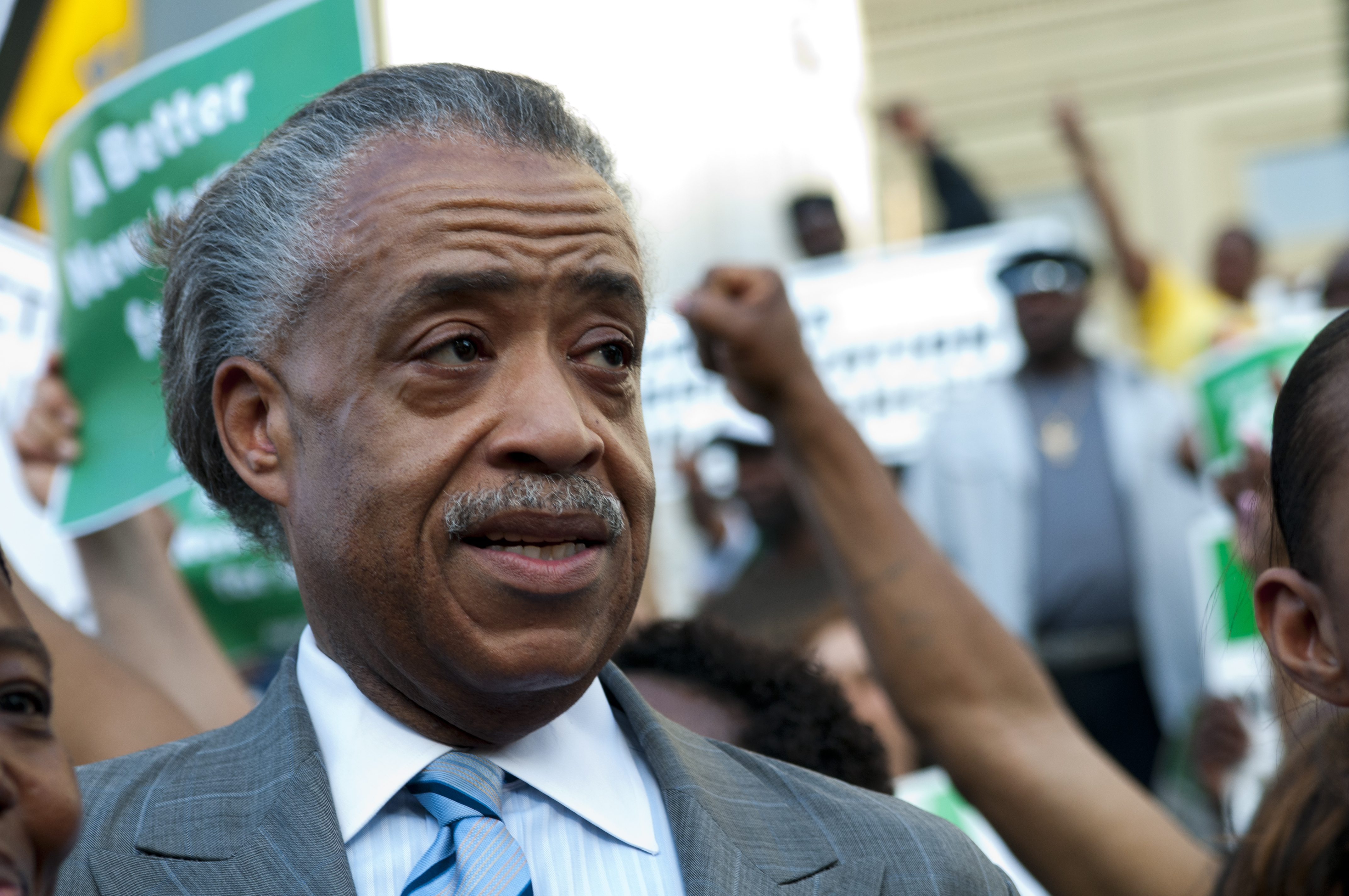This is a photograph capturing the Reverend Al Sharpton at a rally or protest event. He is the primary focus of the image, standing just left of center and appearing to speak passionately. Sharpton is dressed in a striped suit, shirt, and tie. The background is bustling with activity, though the figures there are out of focus. People behind him are energetically pumping their fists in the air, signifying a moment of collective action. Among the blurred signs, one reads partially "A Better, New," though the rest of the text is unclear. One individual wearing a white jacket over a medium blue shirt and a necklace with a large gold medallion stands out. Additionally, there is a green sign with white lettering in the mix. The backdrop includes African American individuals, and towards the right edge of the photo, there's a partial view of an African American woman's head. The color palette of the image spans black, white, gray, brown, green, yellow, and various shades of blue. The origin of the photograph is ambiguous, as it could have been taken by either a bystander or a professional photographer.